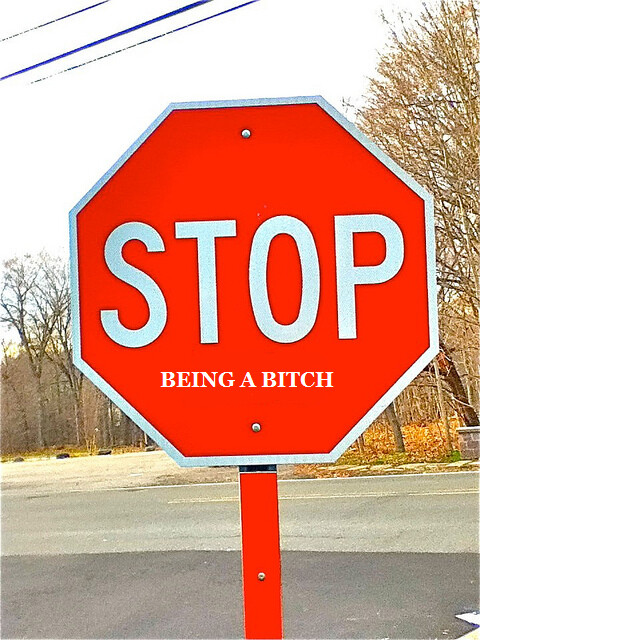In this detailed photographic image, we observe an octagonal red stop sign with bold white text reading "STOP." Below, in smaller white caps-locked font, it says "being a bitch," either added digitally or as a physical sticker. The sign appears relatively new, mounted on a red metal pole, possibly covered with a red strip. The scene is set in a somewhat rural environment with unkempt surroundings, characterized by barren trees devoid of leaves, fallen foliage, and mixed gray pavement. The background reveals an empty lot and a road transitioning from dark to light gray, flanked by a cement wall or partition on the right. Additionally, power lines stretch across the top left corner against a predominantly clear sky with a few dark blue streaks. The lighting and shadows suggest the photo was taken early in the day.